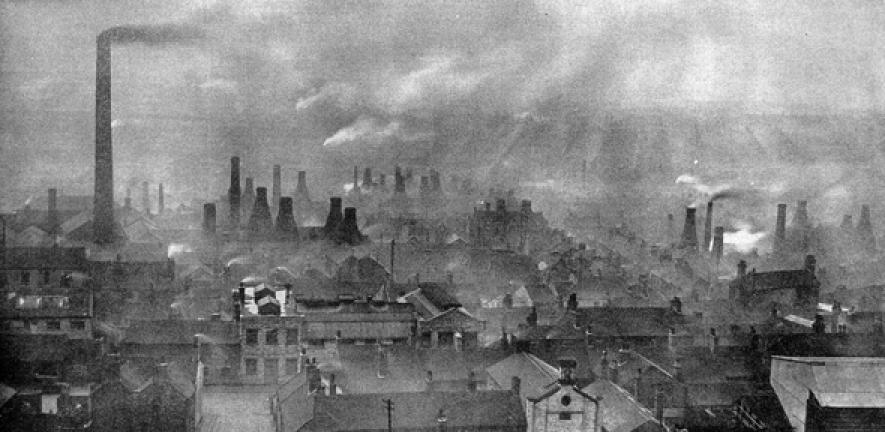This image, possibly from the 1800s, depicts a dark, cloudy, industrial cityscape, reminiscent of old London. The black and white, grainy photograph captures a central factory with a towering smokestack on the left side, emitting thick black smoke into a sky already heavy with pollution. Surrounding the main smokestack are numerous smaller smokestacks and industrial furnaces, further contributing to the smoggy atmosphere. The scene includes several buildings, some with visible chimneys, and a notable white building with a rolled-down gate positioned in the foreground. The rooftops of these structures are predominantly dark, save for one white roof among them. The overall picture conveys a sense of an old, bustling industrial environment, shrouded in the gloom of smoke and clouds.